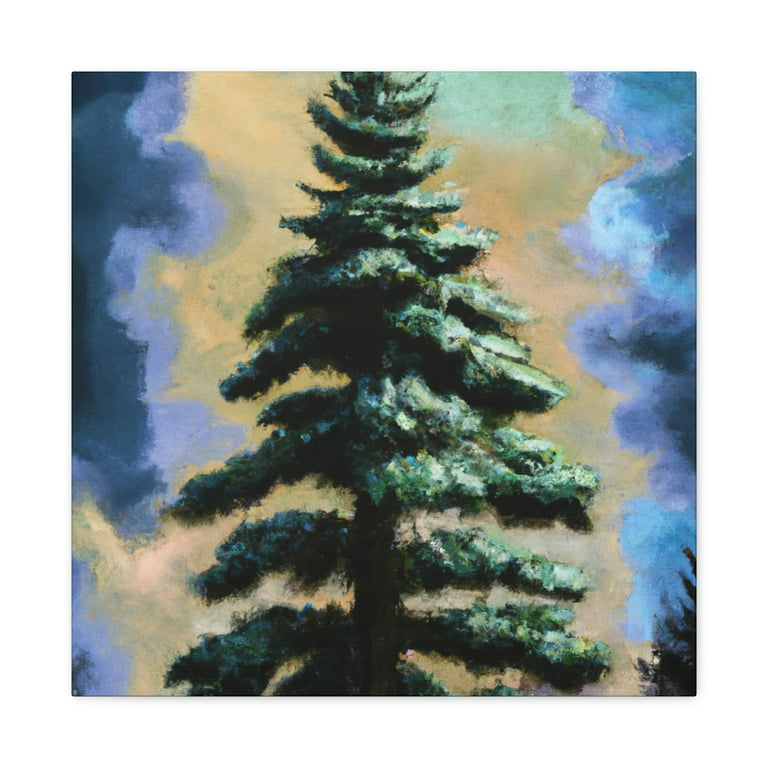This painting features a slender and tall evergreen tree, extending beyond the boundaries of the canvas. The tree, depicted with clear, distinct branches, is enveloped in green leaves or needles with snow subtly dusting its limbs. The lower branches reveal gaps that diminish as the branches ascend and taper. 

The background is a striking blend of a yellowish sky surrounded by dark clouds and shades of light blue, teal blue, mauve, medium blue, dark blue, and black, creating a vivid, contrasting night sky. A light beige halo effect outlines the tree, enhancing its prominence against the captivating sky. Additionally, there is another tree subtly appearing at the bottom right, adding depth, while a small peak of a branch is visible at the bottom left. The brush strokes are loose, contributing to the ethereal atmosphere of the smoke-like, multicolored background.